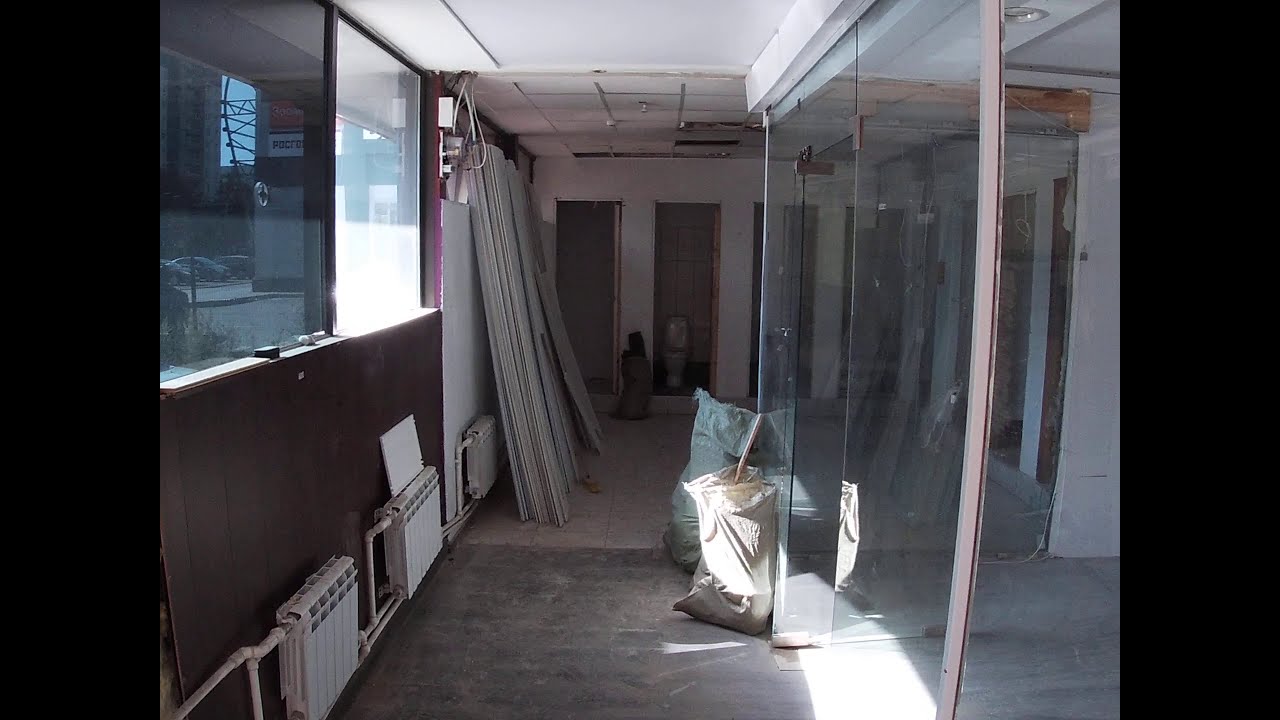This photograph captures the interior of a building, specifically a hallway that seems to be under construction or renovation. On the left side, there is a brown wall extending into a white wall, lined with radiators near the floor and stacked with building materials like white sheets. Above this, two windows let light into the space: the left window is somewhat clear, revealing a distant view of parked cars and buildings, while the right window is more opaque, offering a blurred glimpse of structures behind it. In the middle of the left section, hanging windows allow partial visibility into the exterior scene. The right side features a glass enclosure area, possibly a room with glass walls, with large white and blue sacks propped against it. The flooring throughout is gray. Toward the back of the hallway, the scene is dominated by four brownish vertical doors, and just before reaching the far-right edge, two more vertical doors are visible against a white wall. In the distant background, a small doorway appears to lead to a restroom, partially visible with three stalls, one of which contains a toilet. The overall atmosphere suggests a space in transition, characterized by its construction materials and unfinished appearance.